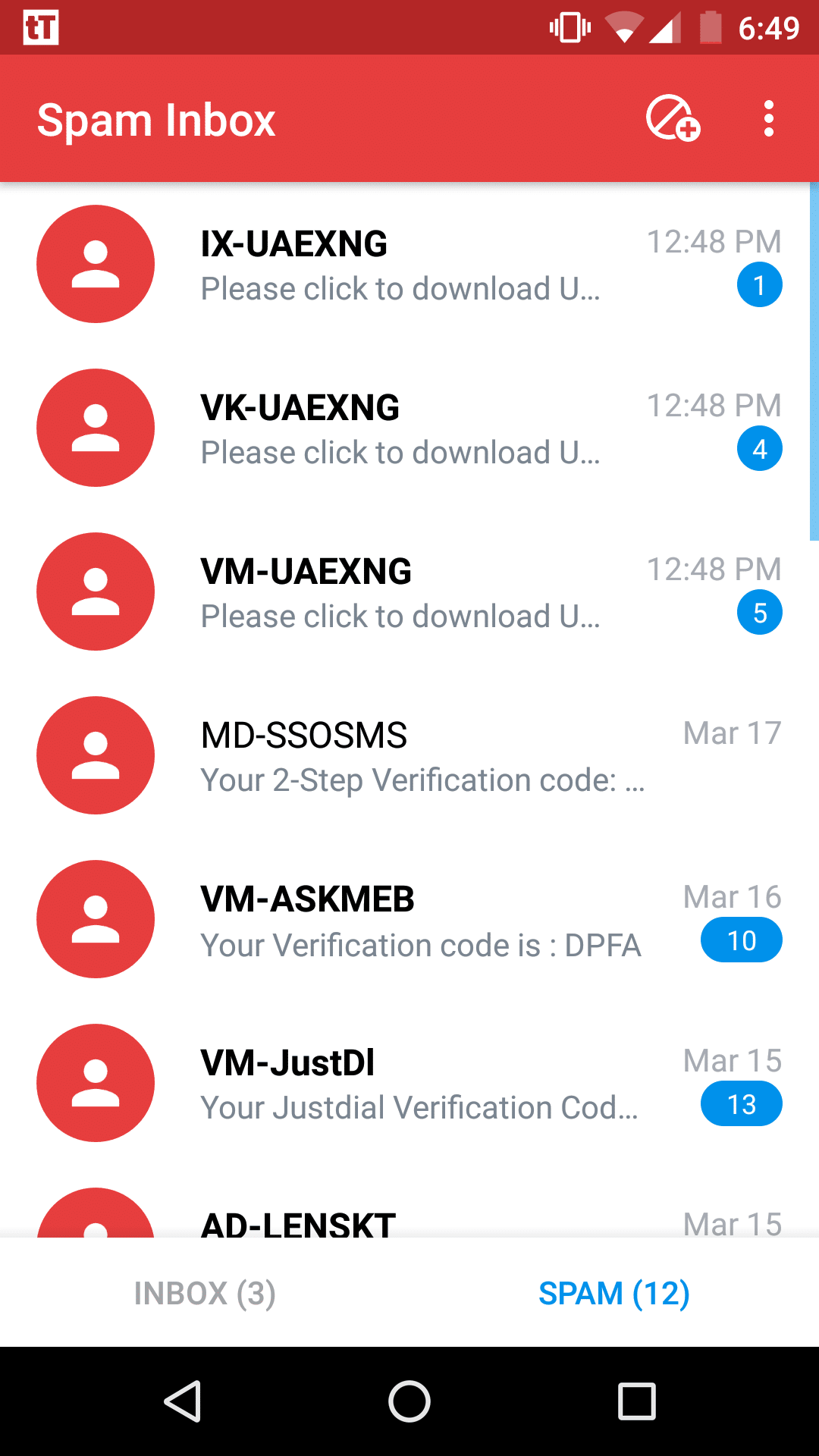**Caption:**

A detailed view of a smartphone screen displays various notifications and system statuses. 

At the very top, on a maroon banner, there are two white squares: one with a small lowercase "t" and the other with an uppercase "T." Next to these, an icon indicating the phone's vibration mode is activated, showing tiny vibration lines on each side. Further along, the Wi-Fi signal is very weak, while the network signal is nearly full. The battery icon is mostly red, indicating it is almost empty, with just a small red line remaining at the bottom. The current time is displayed as "C649" in the top right corner.

Below this, on a red background, the words "Spam Inbox" appear in white text. Adjacent to "Spam Inbox" is a small circle with a line through it and a plus sign, presumably a block option. 

The list of received spam messages includes:
1. "IX-UAEXNG, please click to download you..." received at 12:48 PM, marked with a blue circle containing the number 1.
2. "VK-UAEXNG, please click to download you" received at the same time, 12:48 PM, marked with a blue circle containing the number 4.
3. "VM-UAEXNG, please click to download" also received at 12:48 PM, marked with a blue circle containing the number 5.
4. "MD-SSOSMS, your two-step verification code" from March 17th, without any blue marking.
5. "VM-ASKMEB, your verification code, DPFA" from March 16th, marked with a blue tab containing the number 10.
6. "VM-JUSTDI, your just-dial verification code" from March 15th, marked with a blue tab containing the number 13.
7. "AD-LENSKT" from March 15th, although the full message and blue tab information are obscured.

This detailed snapshot provides an intricate look at the phone's status indicators and the overwhelming spam notifications cluttering the inbox.